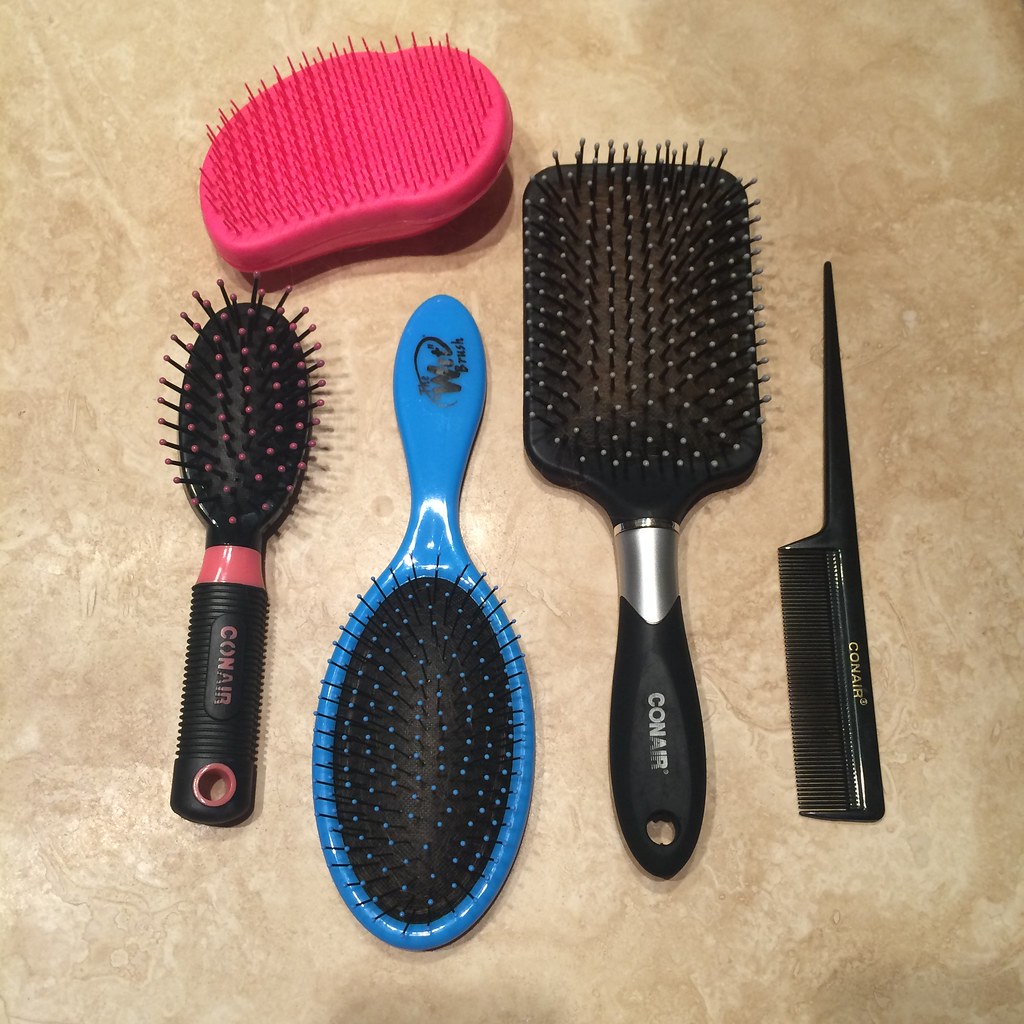The square-oriented color photograph features an overhead view of a collection of hair brushes and combs, organized meticulously on a formica-style surface with a marbled, brownish-tan pattern. The central arrangement includes four items laid out alternately: the first is a black brush with pink detailing, its handle pointing down, followed by a blue plastic brush with its handle pointing up. The third item is another black brush, rectangular with a silver band and the Conair logo, oriented with its handle pointing down. The fourth item is a black plastic comb, also bearing the Conair brand in gold, with its handle directed upwards. Above this row, slightly to the top left, is a bright pink, handheld pet brush, devoid of a handle and shaped like a half-cut potato, with its bristles facing upwards. The layout creates a visually appealing alternating pattern, showcasing a variety of brush and comb designs, underscored by brand uniformity in the Conair-labeled items.